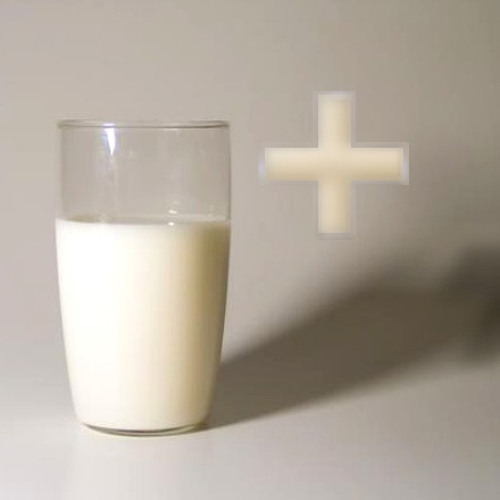The image captures a simple yet striking scene set against a cream-colored background. At the center, there is a cylindrical glass of milk, filled to about two-thirds capacity. The glass slightly widens towards the top and features a light reflection around its rim, emphasizing its transparency. A shadow extends from the right side of the glass, grounding it in the image. Adjacent to the glass, near the top where the milk level ends, there is a plus sign or cross symbol. This symbol, outlined in white, mimics the color of the milk with a beige-filled interior, blending subtly into the background. The overall composition, with its minimalist elements and delicate color palette, could suggest an advertisement, highlighting purity or health.